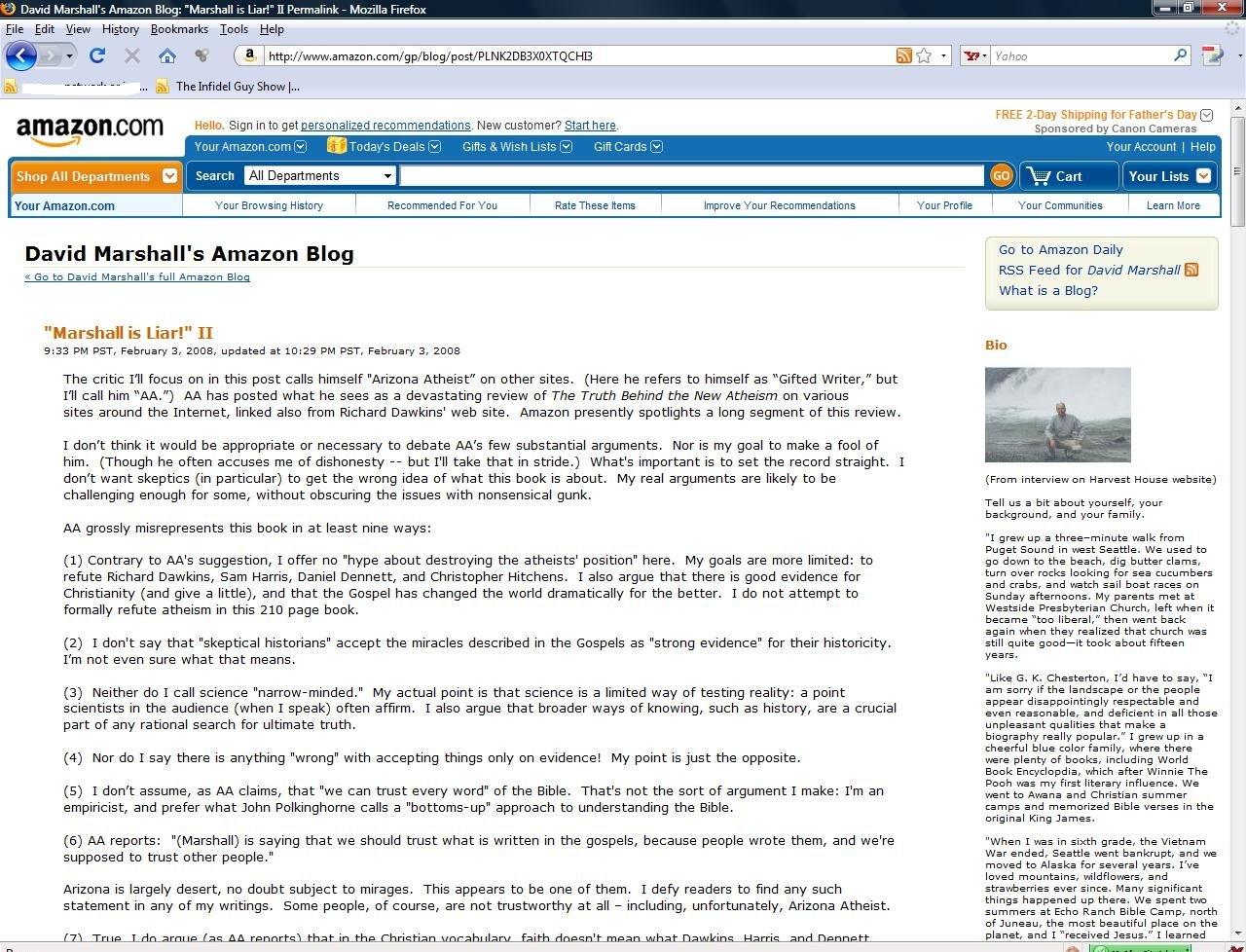David Marshall's Amazon blog, "Marshall is a Liar," is displayed prominently at the top within a Firefox browser window. The screen contains several browser interface elements such as the File, Edit, View, History, Bookmarks, Tools, and Help menus. There are icons for Lecture, Video, Refresh, and others leading to various functionalities including navigating back to the homepage and refreshing the page.

The URL bar shows "amazon.com/gps/blog/post/blk2db3x0xtqch3" and an orange RSS feed icon is visible. To the right, there are options to access the Infidel Guy show and to sign in for personalized reviews and recommendations. New customers are addressed, promoting features such as free 2-day shipping, fraud-free services, and responsible accounting.

Further down, Amazon highlights today's deals, gift options, wishlists, gift cards, and child-related departments. A search bar is available along with browsing history and tailored purchasing recommendations. There's an invitation to approve recommendations, view your profile, and engage with communities.

In the background is a nostalgic memory: a group of friends spending Sunday afternoons together, digging for butter clams at the beach, and turning over rocks to find sea cucumbers and crabs. They visited a church on the west side, made a journey to Liverpool, and despite some tiredness from the trip, appreciated the good experience at the church.